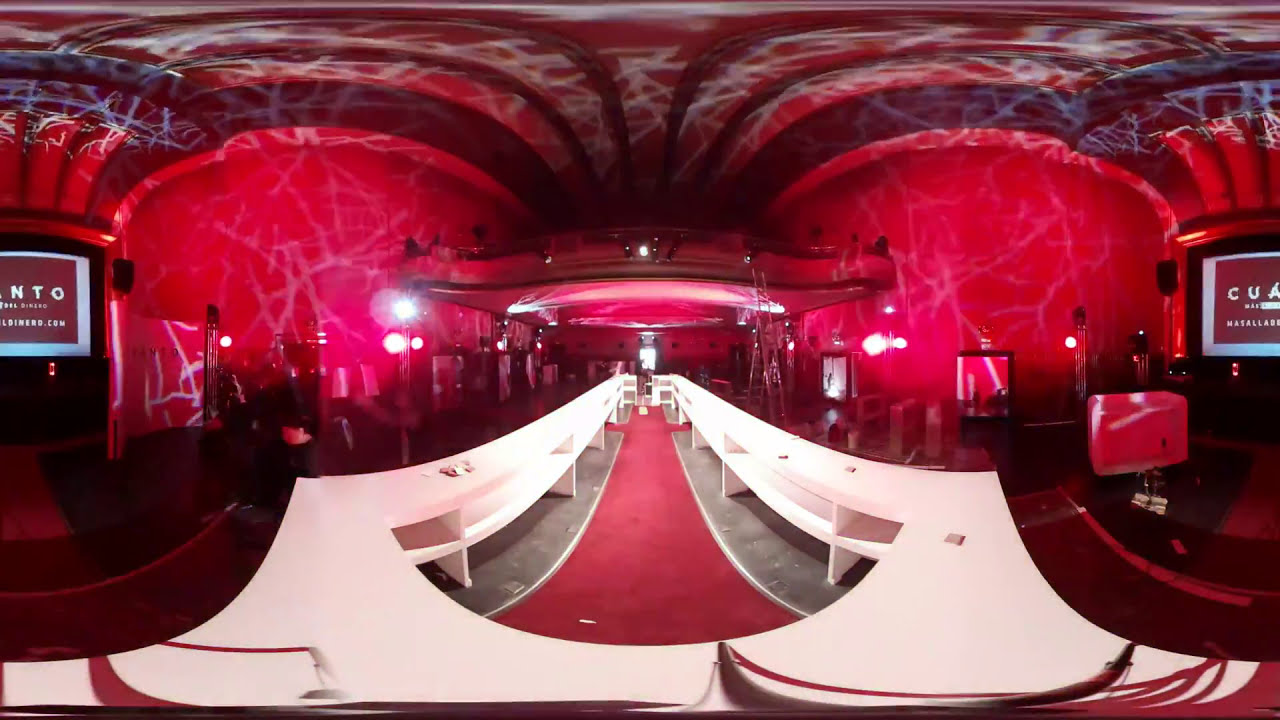The image depicts a strikingly modern, room that could be a bar or nightclub. Dominated by a vivid red color scheme, the room features an expansive red carpet running down its center. On either side of the carpet, there are sleek white wooden-designed shelves, contributing to its contemporary aesthetic. The walls and ceiling are predominantly red, possibly enhanced by dynamic, dramatic lighting that creates a romantic, club-like ambiance. Intriguingly, the ceiling features alternating red and white stripes with circular white patterns. At the center of the room is a large, circular bar table, reminiscent of a bar area yet to be stocked, where bartenders would serve from the middle. The lighting includes spherical fixtures on the walls, adding to the innovative design. Two large TV screens hang prominently, displaying messages partly obscured, ending with "NTO" and "something.com". The entire setting appears very futuristic and possibly captured using a virtual reality camera, adding to its immersive and slightly surreal illusion with reflective, almost electric backdrops that blend both halves of the room seamlessly.